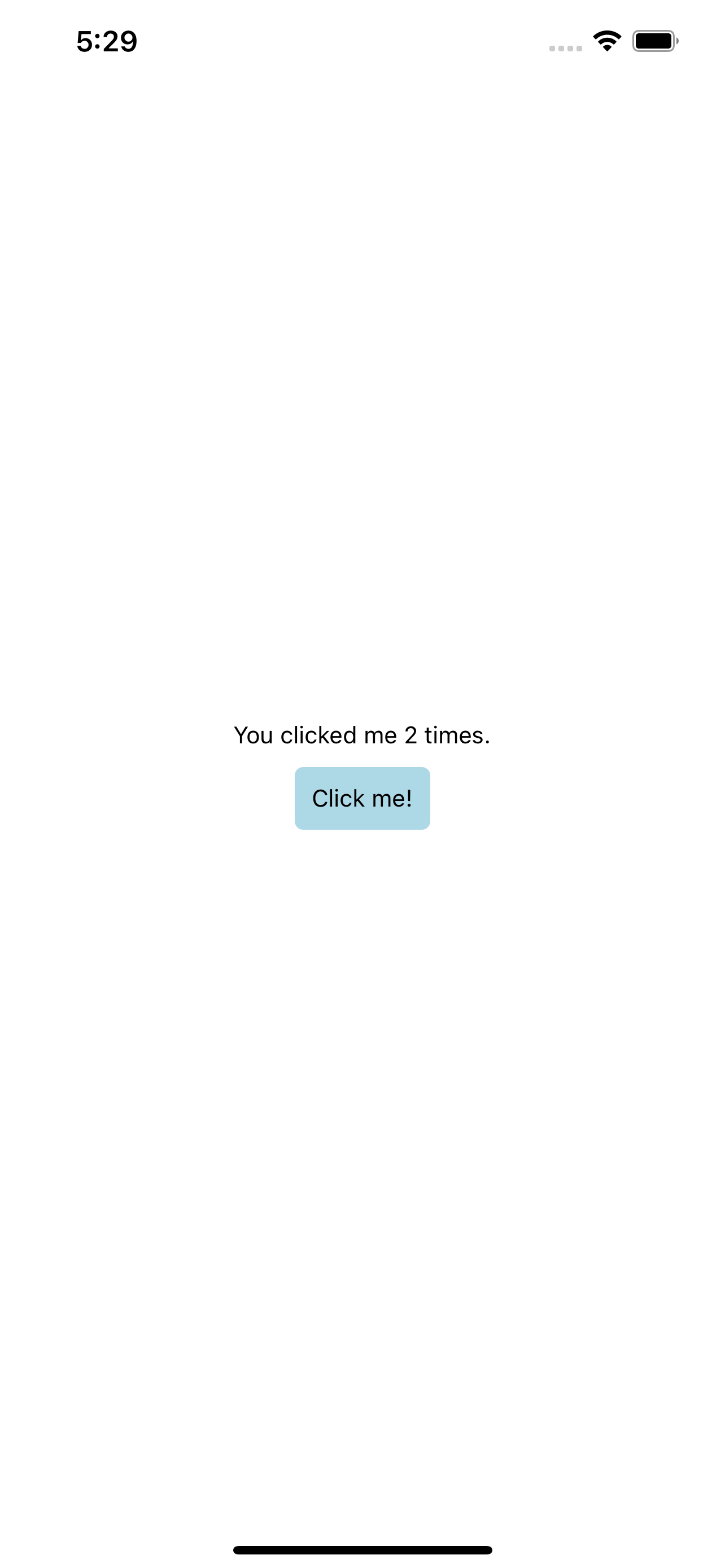**Caption:** A screenshot of a smartphone display shows a predominantly white background with various interface elements. At the top of the screen, the time is displayed as 5:29. To the right, four dots and an inverted cone-shaped icon indicate a strong internet connection, represented by three fully filled bars. Adjacent to these indicators is a battery icon showing a fully charged battery.

Centrally positioned on the screen, small black text reads "You clicked me two times," accompanied by the numeral "2." Beneath this text, there is a small, light-blue rectangular button with black text that reads "Click me!" Towards the very bottom of the screen, a long, dark-black bar extends across approximately two-thirds of the middle section. The overall design of the screenshot is simple and minimalistic, with clear emphasis on interactive elements and status indicators.